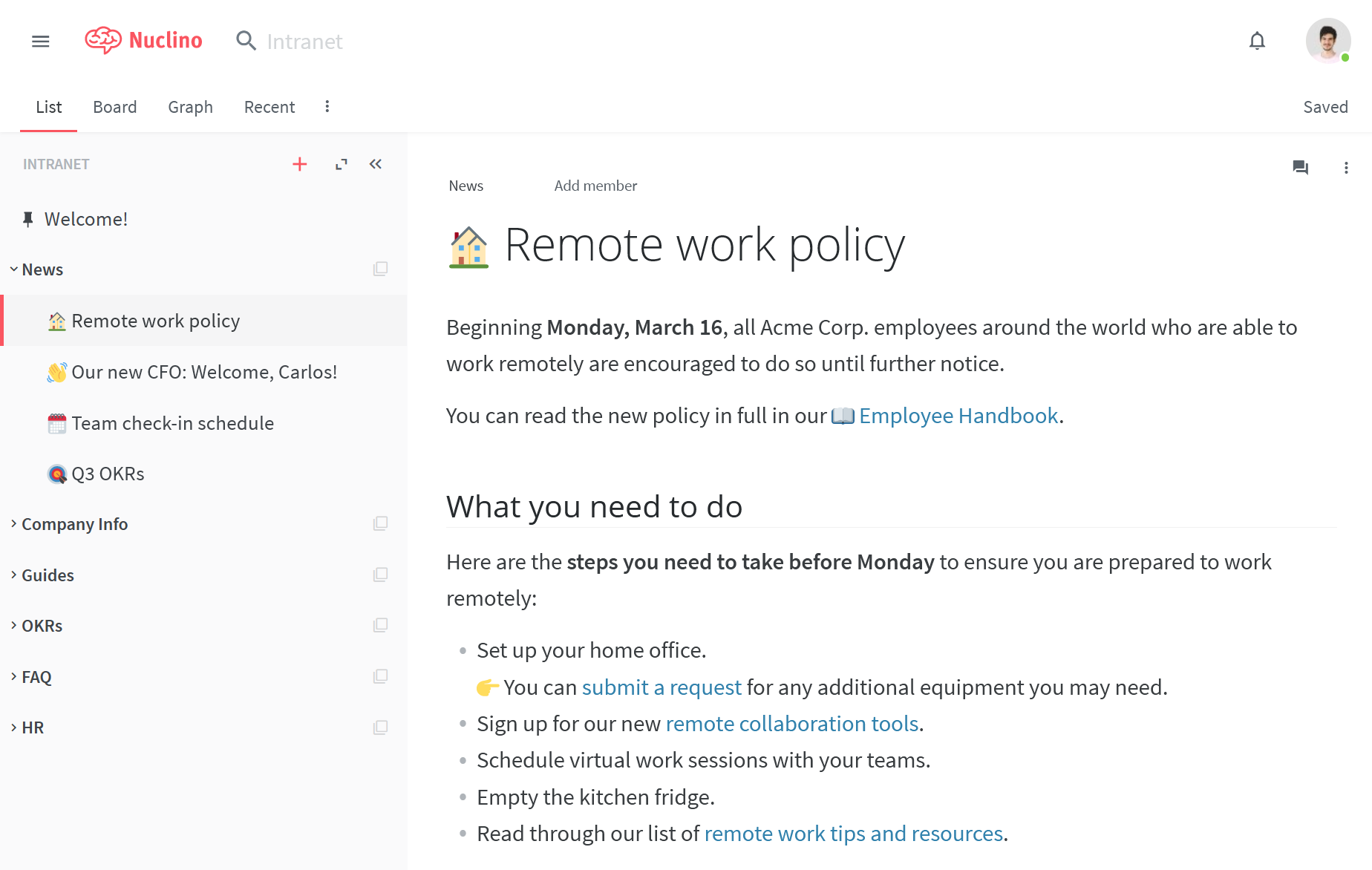This image is a landscape-oriented screenshot taken from a website's internal page, with the proportions typical of a display on a computer or laptop screen. The predominant background color is white. At the top of the page, a white header holds a hamburger menu on the left, and next to it, in black and red text, is a logo resembling a brain and labeled "Nuclino". Adjacent to the logo is a white search box with a gray magnifying glass icon and the placeholder text "intranet." Further to the right, there is a notifications icon and an avatar of a person with black hair set against a gray circular background, accompanied by a green dot indicating that they are currently active.

Below the header, there are several navigational options labeled "List," "Board," "Graph," and "Recent," with "List" being highlighted in blue or underlined in red. To the right of these options is the word "Save."

The main content area begins with the word "Intranet" displayed within a gray portrait-style box, followed by a welcome section pinned at the top. A news drop-down menu features updates titled "Remote Work Policy," "Our New CFO," "Team Check-in Schedule," along with other unspecified options. Additionally, there are expandable sections labeled "Company Info," "Guides," "OKRs," "FAQs," and "HR."

To the right side of the content, there is a house icon next to the heading "Remote Work Policy." The accompanying text states: "Beginning Monday, March 16th, all Acme Corp employees around the world are able to work remotely and are encouraged to do so until further notice," followed by a more detailed description underneath.